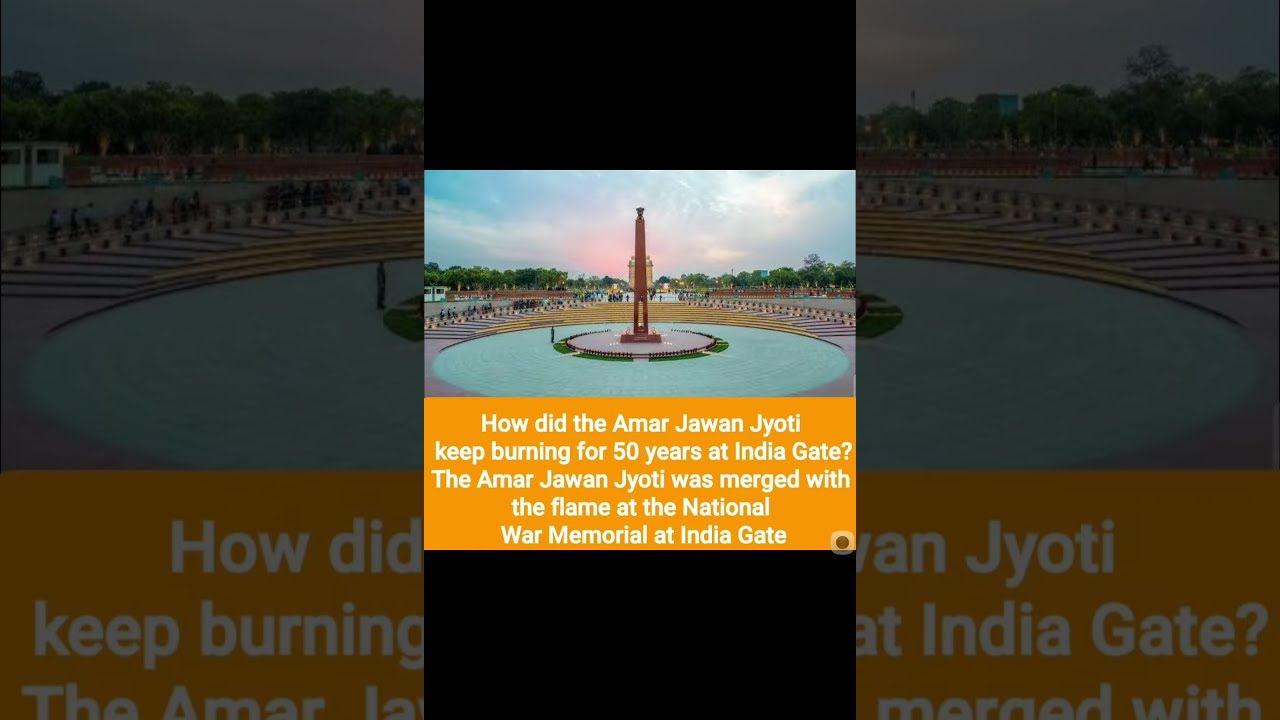This image depicts a vertically oriented scene focused on a central, cylindrical monument, likely a fountain, with a red tall and thin section in the middle atop a brown base. Surrounding the monument at its base appears to be blue water, encircled by concrete. The image is bordered by black rectangles on the top and bottom, giving it a cinematic feel. Both the left and right sides show blown-up segments of the main picture, mirroring each other by displaying parts of the memorial, some writing, and the background.

In the middle section of the image, just above the bottom black rectangle, there's a prominently displayed caption framed within an orange strip that reads: "How did the Amar Jawan Jyoti keep burning for 50 years at India Gate? The Amar Jawan Jyoti was merged with the flame at the National War Memorial at India Gate." This text is in white against a mustard-colored background.

The central part of the image includes a view of a blue sky dotted with clouds, a tree-lined horizon, and what resembles a parking area with indistinct structures. The central fountain itself shows no water flowing, and the main focus is sharply contrasted against a larger background image that is gray-toned and slightly obscured by the central visual elements.